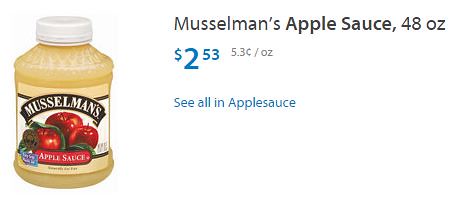This advertisement for Musselman's applesauce showcases a 48-ounce plastic jar with a white, breakaway safety seal cover, set against a white background. The jar features a green label with bold white "Musselman's" text, accompanied by images of three vibrant red apples with green leaves, and a smaller red label indicating "applesauce." The price, $2.53, equating to 5.3 cents per ounce, is displayed in aqua blue font to the right of the jar, with an invitation to "See all in applesauce" directly below in blue-green font. The advertisement emphasizes a clear and detailed view of the product, highlighting the traditional round design of the Musselman's applesauce jar.